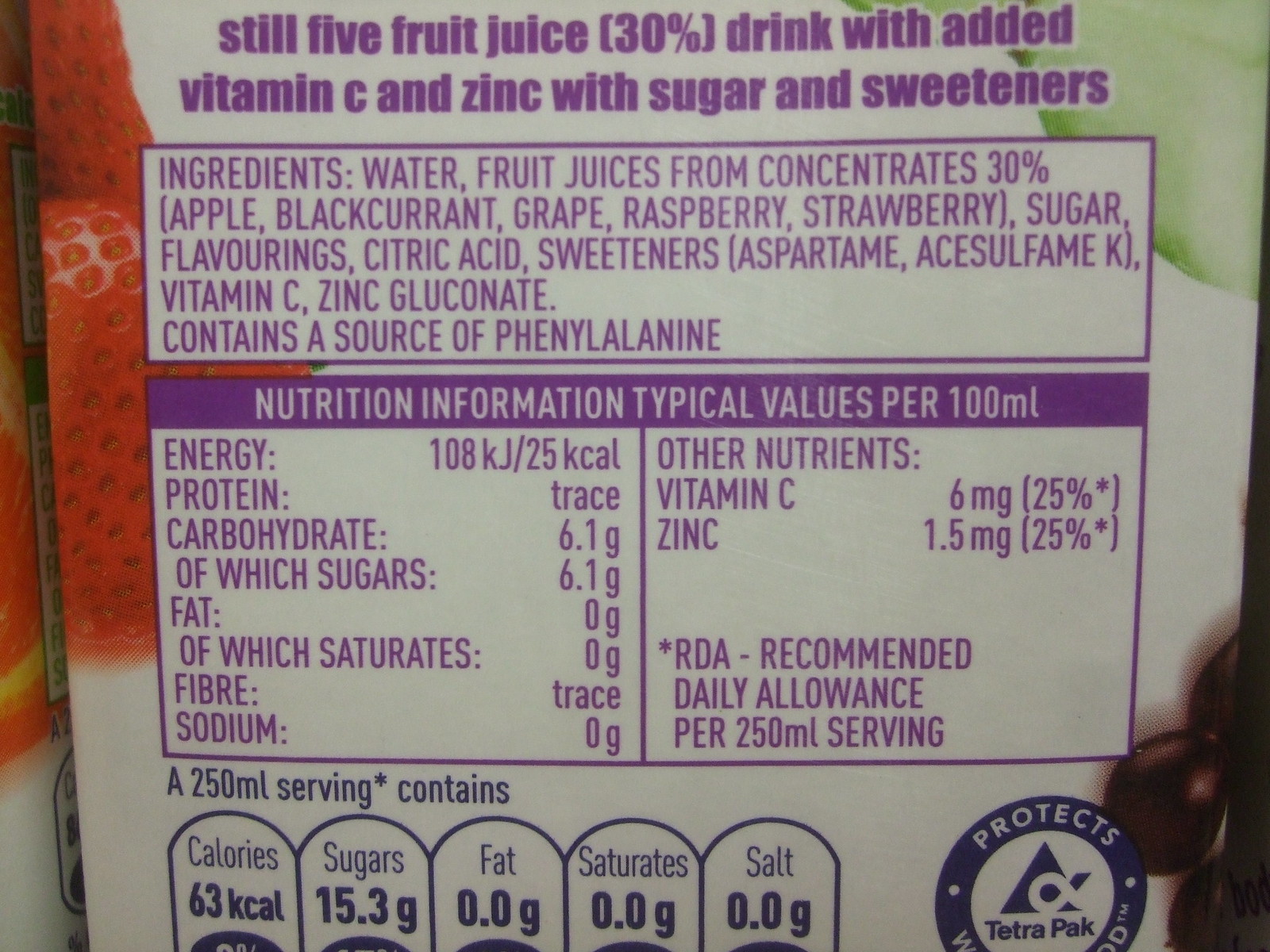This image is a close-up photograph of the back of a fruit juice drink container against a white background, featuring the ingredients list and nutritional information. At the top, written in purple text, it reads, "Still 5 Fruit Juice, 30% drink with added Vitamin C and zinc with sugar and sweeteners." The background features partially visible graphics of strawberries on the top left, blackcurrants on the bottom right, and a mix of other fruits. The ingredients box lists water, fruit juice from concentrate (30%) including apple, blackcurrant, grape, raspberry, and strawberry; sugar, flavorings, citric acid, sweeteners such as aspartame and acesulfame K, Vitamin C, and zinc gluconate. It also contains a notice about phenylalanine. The nutrition box details the typical values per 100 milliliters, highlighting energy, protein, carbohydrates (of which sugars), fat (of which saturates), fiber, sodium, Vitamin C (6mg, 35% RDA), and zinc (1.5mg, 35% RDA). The bottom section outlines the energy value and the amounts of calories, sugars, fats, saturates, and salt per 250ml serving: 63 kJ, 15.3g sugars, 0g fats and saturates, respectively.